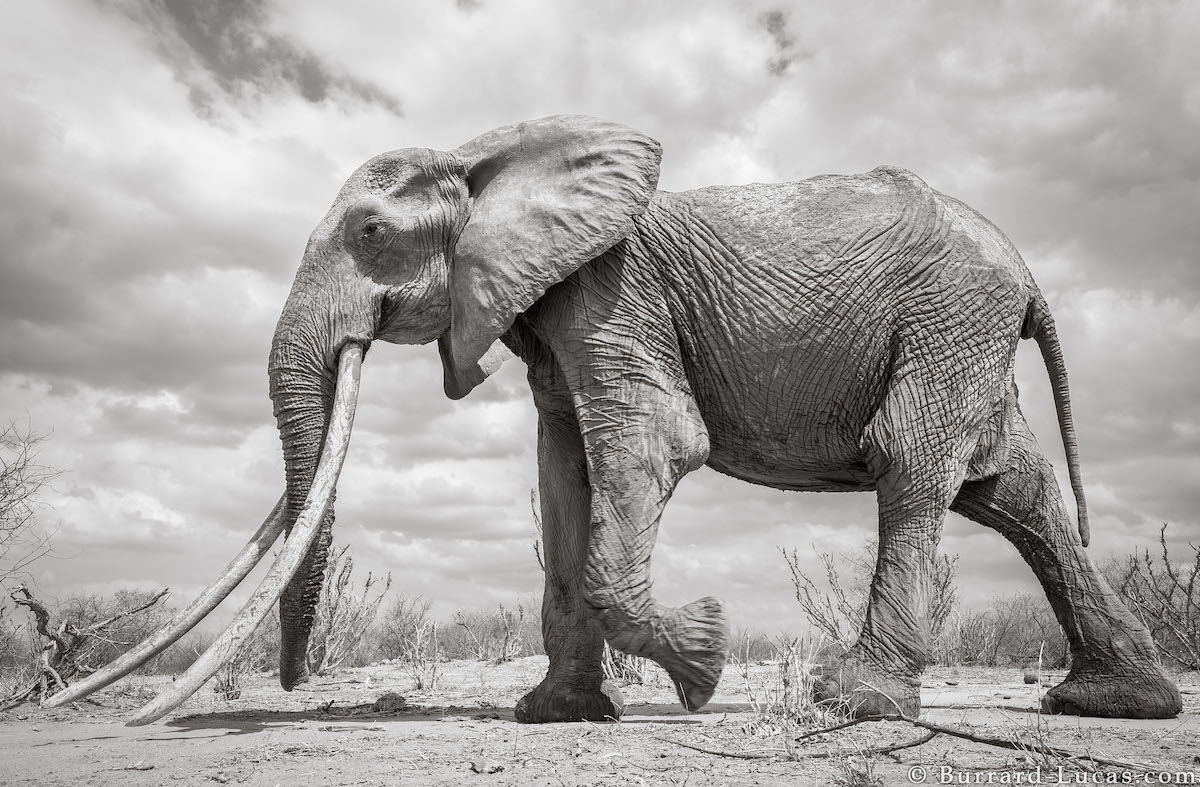An evocative black-and-white photograph, potentially the work of professional photographer Burrard Lucas, captures an aged elephant traversing a dry, barren landscape. The copyright mark in the bottom right corner credits burrard-lucas.com. The elephant is presented in a side profile, with exceptionally long tusks nearly touching the cracked, arid earth. Its wrinkled skin and frail frame suggest advanced age and possible undernourishment. The elephant’s front left foot appears to be mid-step, while its ears lie back and tail hangs down, illustrating a dynamic moment in its stride. Taken from a low angle, the shot accentuates the imposing yet vulnerable presence of the majestic creature. Sparse scrubby vegetation dots the background, set against a uniformly overcast sky, indicating a savanna setting in a season of drought or desolation. The photograph exudes a sense of raw, timeless beauty amidst the struggle for survival.